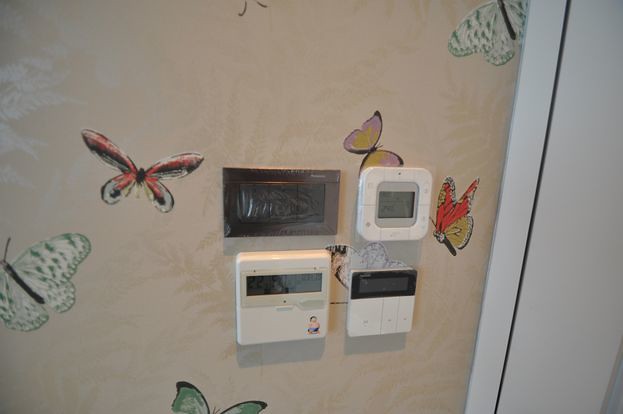The image showcases a tan wall adorned with a leaf-patterned background and decorated with multiple butterfly stickers in vibrant shades of green, red, purple, yellow, and black. Central to the composition are four distinct thermostats arranged in a grid. The top left thermostat is a dark copper-colored rectangle, complemented by a white thermostat with a gray screen beside it. On the lower row, the left side features a larger white square thermostat that has a small sticker on its bottom edge, and next to it is another white thermostat with a black and gray screen. Surrounding these devices, butterfly stickers add a splash of color, with two butterflies perched to the right of the thermostats and three on the left. Additionally, two butterflies are positioned at the top, one partly visible in the corner and another showing only its antennae descending from the top edge of the picture. To the right of the thermostats, a white door or wall completes the scene.